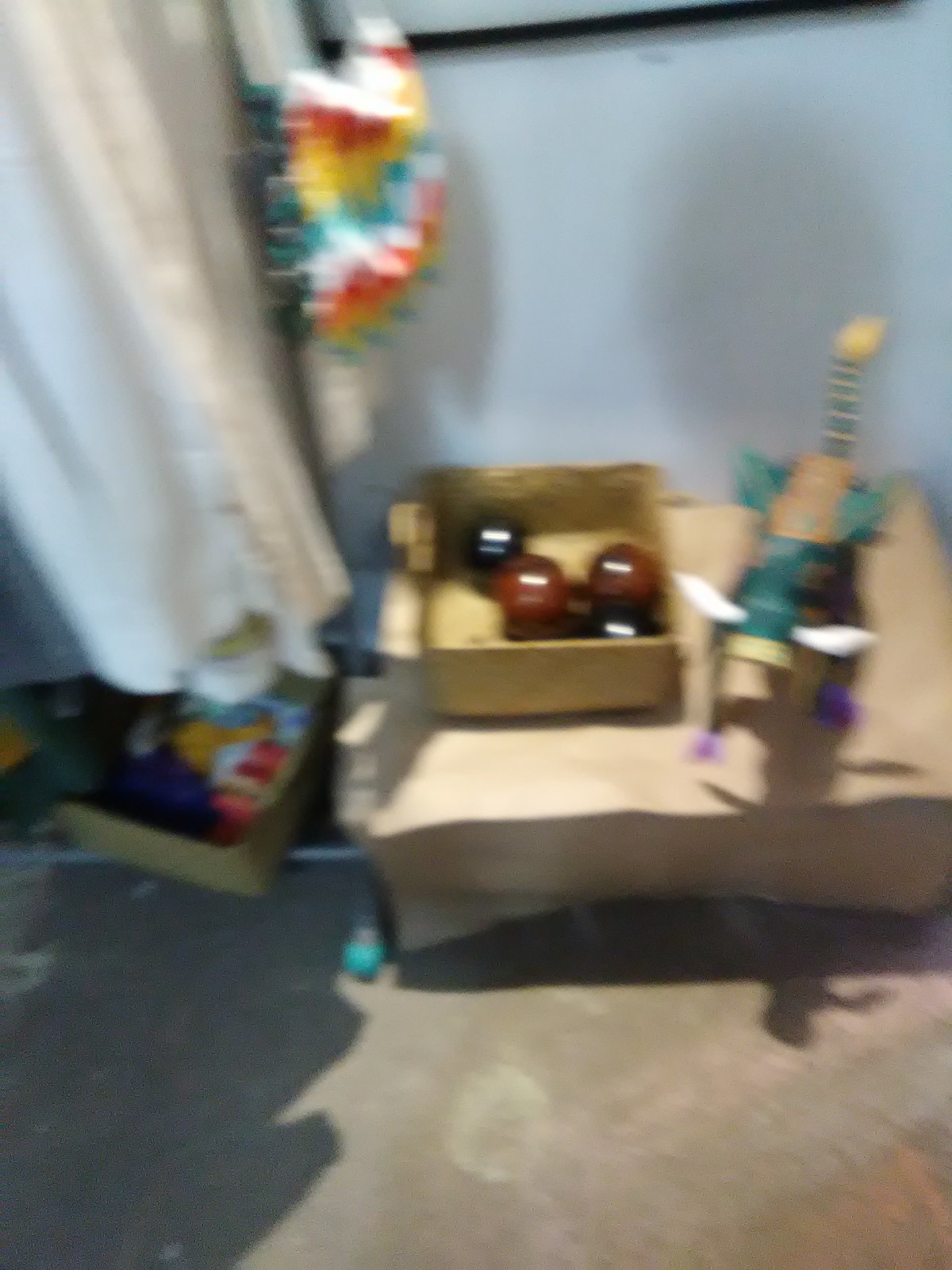The image depicts a cozy room with blue walls, featuring a curtain that either covers a window or divides the space. In the room, a wooden bookcase or shelf is prominently displayed, holding a box filled with brown and black balls. A guitar with a striking turquoise base rests nearby. The floor is carpeted in a soft tan to beige, adding warmth to the setting. Scattered across the floor are various toys, suggesting a playful atmosphere. A colorful bag with white, red, yellow, and blue stripes hangs from a rack, possibly adorned with beads, adding a touch of whimsy to the scene.